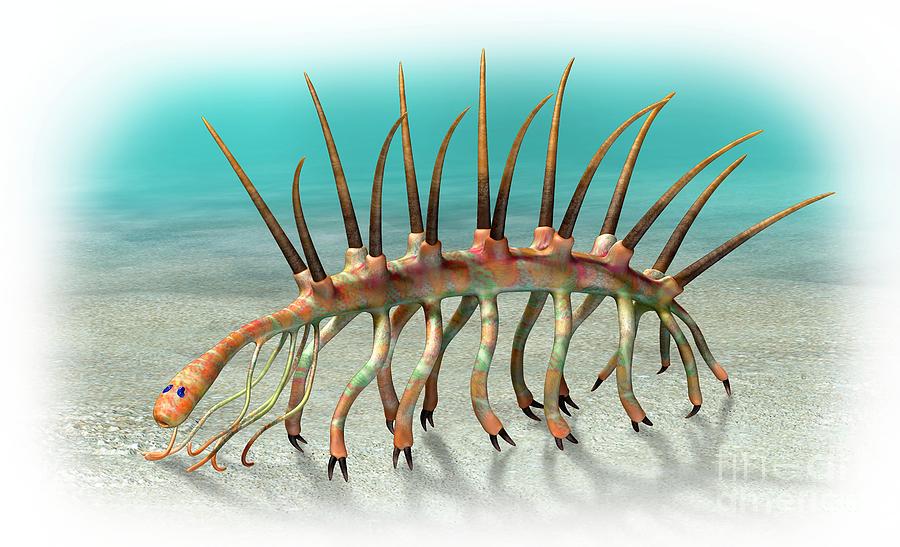The image depicts a cartoony, video game-style sea creature, set against a bright blue sea floor background that fades out around the edges in an oval shape. The lower right-hand corner features an indiscernible watermark. The creature dominates the oval space and presents an alien, bug-like appearance, with a very long and thin body that is subtly striped in orange and green hues. It has a cylindrical head with blue eyes and a mouth, and is adorned with 14 spines along its back, somewhat resembling a porcupine’s quills.

The creature has a total of 14 legs, each ending in spiny tips, and varying between one and two claws per leg. Additionally, it features six long tentacle-like feelers protruding from its front. The body structure appears skeletal or framework-like, emphasizing its spiny and delicate nature. While it might look reminiscent of a land porcupine due to its spines, it lacks the fleshy body, making it appear more skeletal or alien. The background, with its tan sea floor and teal water, firmly places this fantastical creature in an underwater setting.